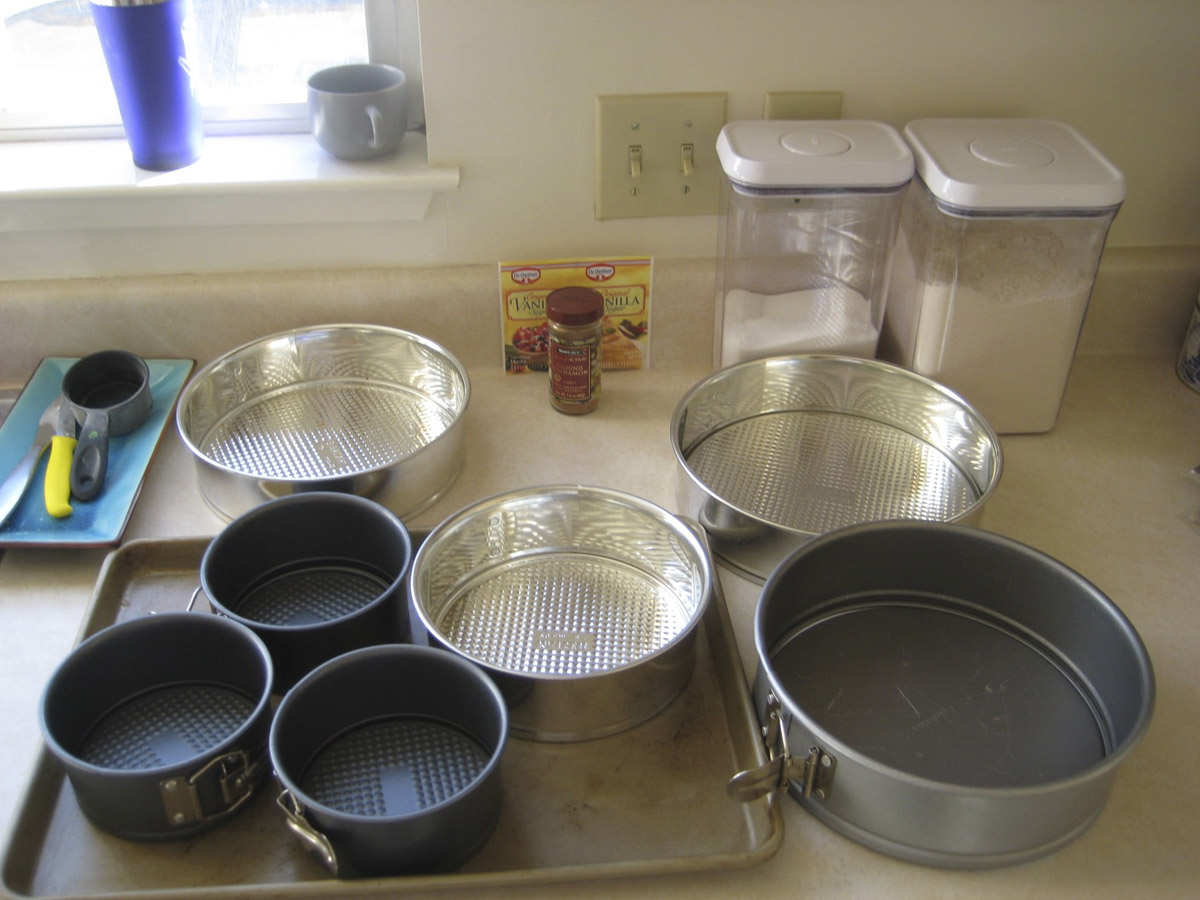The image is a color photograph of a kitchen countertop neatly arranged with various baking pans and utensils. The focal point is a lineup of seven cake pans, most of which are round and have snap-off rims. These pans vary in color and material: three are blue steel, three are shiny white aluminum, and one is dark gray. Some of the pans, particularly the silver ones, feature intricate pattern designs. The countertop itself is a light creamy color. 

In addition to the cake pans, there are other baking-related items visible. A blue dish on the left of the image contains a measuring cup, a knife, and a spoon. Behind the pans, there are containers that likely hold flour and sugar, as well as a small jar possibly containing cinnamon. We also see a cookie sheet among the items. The top left portion of the image features a windowsill with a blue glass and a gray coffee mug. A wall light socket is visible in the background, adding to the detailed domestic scene.